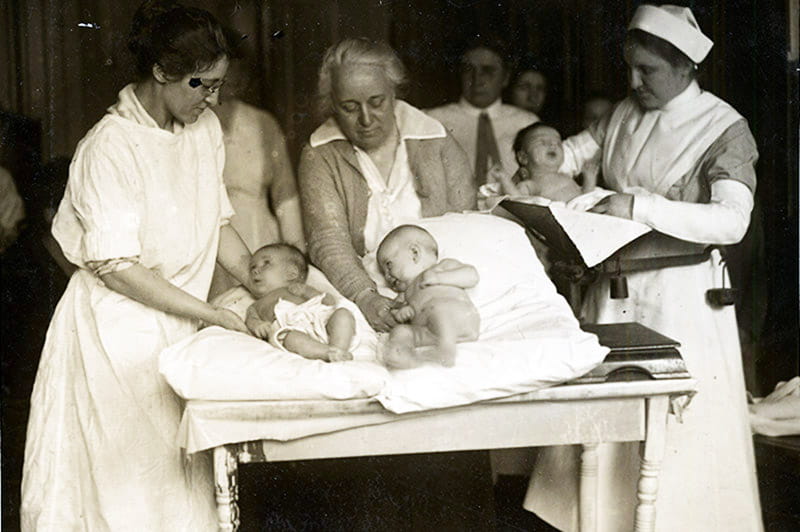This evocative black-and-white photograph, likely taken nearly a century ago, captures a poignant scene involving three women who appear to be nurses. One woman is definitively dressed in traditional nurse's attire, solidifying her role. Each woman cradles an infant, carefully placing them on pillows as if to display them. The babies, dressed only in diapers, are the focal point of this tableau. The surrounding onlookers add a layer of curiosity and speculation to the scene, highlighting its public nature. The nurse on the right seems to be weighing the infant in her care, suggesting a health assessment might be taking place. It's possible the photograph depicts a clinical evaluation of the babies' health before reuniting them with their mothers. Alternatively, the women could indeed be the mothers themselves, proudly presenting their newborns to an eager audience. The image captures a moment of communal interest and tender care, though its exact context remains shrouded in history's mysteries.